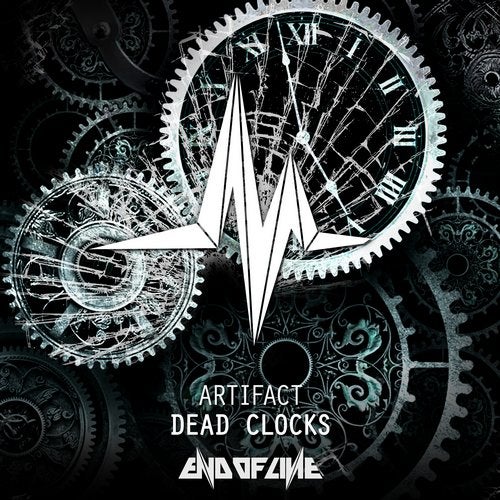The image is a detailed and intricate illustration resembling an album cover due to its square dimensions. The background is predominantly black, creating a stark contrast with the foreground elements. The main focus is on the complex gear work, which appears to depict the inner workings of a clock or watch, featuring interconnected cogs and gears. A prominent gear wheel in the middle upper section has a clock face with Roman numerals and hands indicating a time of two minutes to five. The clock face is encased in broken glass, adding to the texture and theme of decay.

The gears are shaded in light blue, gray, and hints of turquoise, enhancing the mechanical and industrial feel of the image. Among the gears, some have ornate decorations of scrolls, vines, and petals, adding a touch of elegance to the stark mechanical imagery. In the mid-left section, another gear incorporates smaller intricate cogs, all interlocking and contributing to the overall impression of a complex, broken timepiece.

In the lower portion of the image, bold white capital letters read "ARTIFACT," followed by "DEAD CLOCKS." Beneath this, in a thicker, stylized font with exaggerated 'N's, the words "END OF THE LINE" are displayed, with the stylistic elements matching the letter 'M' found within the clock face. This combination of imagery and text strongly suggests the concept of defunct timekeeping devices, reinforcing the speculative notion that this could be an album cover titled "Artifact: Dead Clocks" by a group perhaps named "End of the Line."